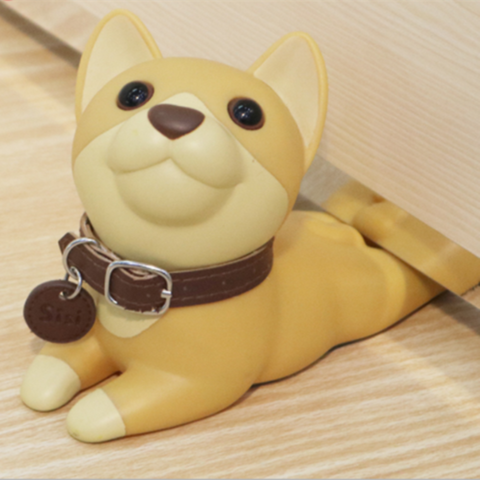This image features a small, detailed statue of a dog, resembling a Shiba Inu, with a distinct light beige or yellowish-tan coat. The dog, possibly made of clay or porcelain, is sitting with its front legs prominently visible, while its hind legs appear to be tucked underneath a piece of furniture, suggesting it could also function as a doorstop. The dog gazes upwards with expressive, big brown eyes and a brown nose. Around its neck, it wears a realistic-looking brown leather collar adorned with a silver buckle and a name tag inscribed with "Sissy." The dog's pointed ears and meticulous details give it an endearing, lifelike quality. The background features a light brown wooden texture, enhancing the warmth and charm of the scene.